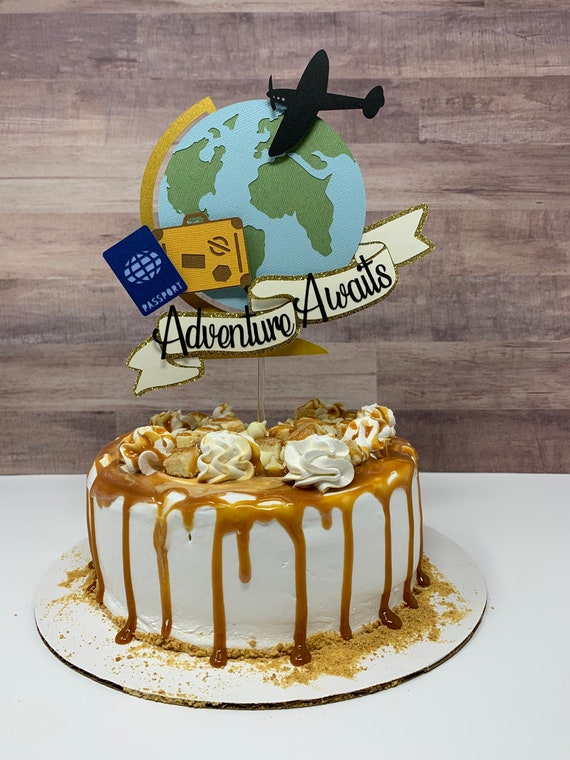This indoor photograph captures a visually appealing and intricately designed cake resting on a light gray or off-white tabletop. In the lower portion of the 5-inch high by 4-inch wide rectangular image, the tabletop forms the base, while the upper portion is dominated by a backdrop of brown wooden horizontal slats.

Centrally positioned on the table is a circular cardboard cake plate, supporting a striking two-tiered cake. The cake, adorned with smooth white frosting, is artistically accented with a rich caramel drizzle cascading from the top and dripping enticingly down the sides. At the base, a sprinkling of graham cracker crumbs adds texture and a touch of rustic charm.

The cake’s top is decorated with delicate dollops of whipped cream, each crowned with a piece of shortbread cookie, further drizzled with caramel. Protruding elegantly from the cake is a thin, clear acrylic straw, which supports an eye-catching cutout: a globe with vibrant green continents and blue oceans encircled by a gold band on the left side, and an image of a black airplane soaring across it.

Adjacent to this globe cutout are illustrations of a blue passport and a brown suitcase, emphasizing the travel theme. Completing this evocative design is a white banner with glittering gold edges and the words "Adventure Awaits" inscribed in black print, adding an inspiring touch to this delectable creation.